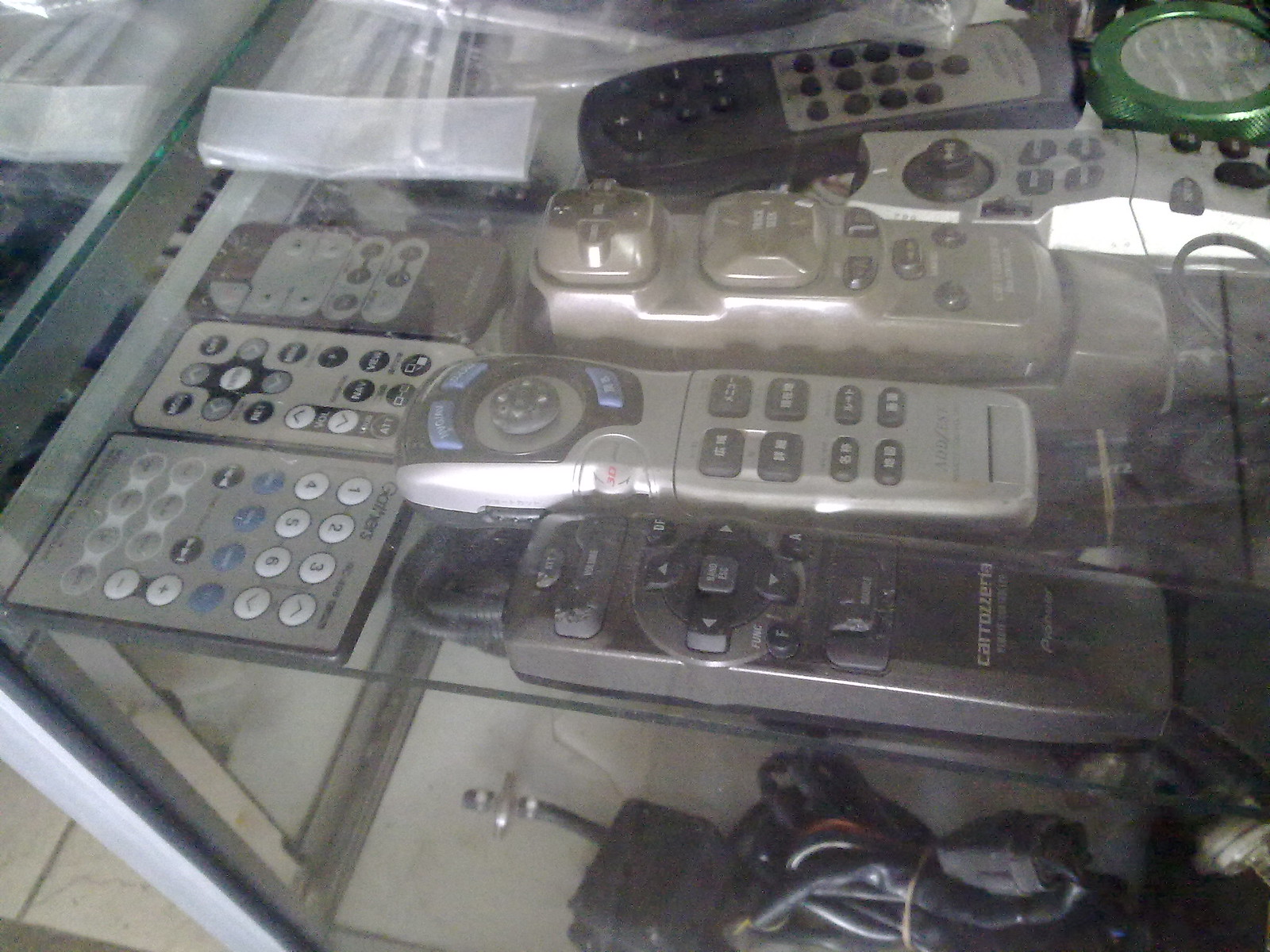The photograph captures an indoor scene featuring a glass display case, typically found in a retail store, presumably a second-hand or thrift store based on the condition of the items. At the top left of the display, there are slimmer, smaller remote controls, possibly for Bluetooth lights or speakers, which are oriented horizontally. The middle section showcases larger, possibly vintage remotes from the late 90s to early 2000s, which may have been used for older appliances like massage pads. Many of these remotes are gray or black with various button colors such as white, blue, and black. The top shelf specifically displays 1980s style used remotes, lying flat, including a light gray one in the foreground, a silver one next to it, and a polished silver one just behind. The image also shows a coiled black cord at the bottom and additional wires, with a silver bar on the left side of the cabinet and a white tile floor visible in the bottom left corner. The image is slightly hazy and out of focus due to light reflections on the glass. In the top right of the case is a green metal object, possibly a lens or cap with a glass center.